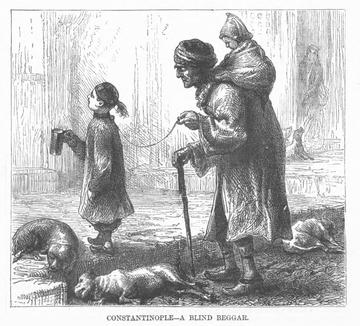This detailed black and white sketch, likely done in pencil or charcoal, is titled "Constable - A Blind Beggar." It depicts a poignant scene: a blind man, hunched over and navigating with a cane, appears in the center of the drawing. He wears a coat with long sleeves and boots visible beneath it, and something is wrapped around his head. Mounted behind his head is a small child, possibly a baby, wearing a pointy hat. 

In front of the man is a young girl with black hair pulled back into a ponytail. Disturbingly, she is attached to him by a leash and holds a cup in her hand, suggesting she is begging for food or money. Below this group, several emaciated dogs lie on the ground, adding to the drawing's bleak atmosphere. The only colors present are shades of white, black, and gray, emphasizing the somber mood. A gray bar at the bottom of the image bears the caption: "Constable - A Blind Beggar."